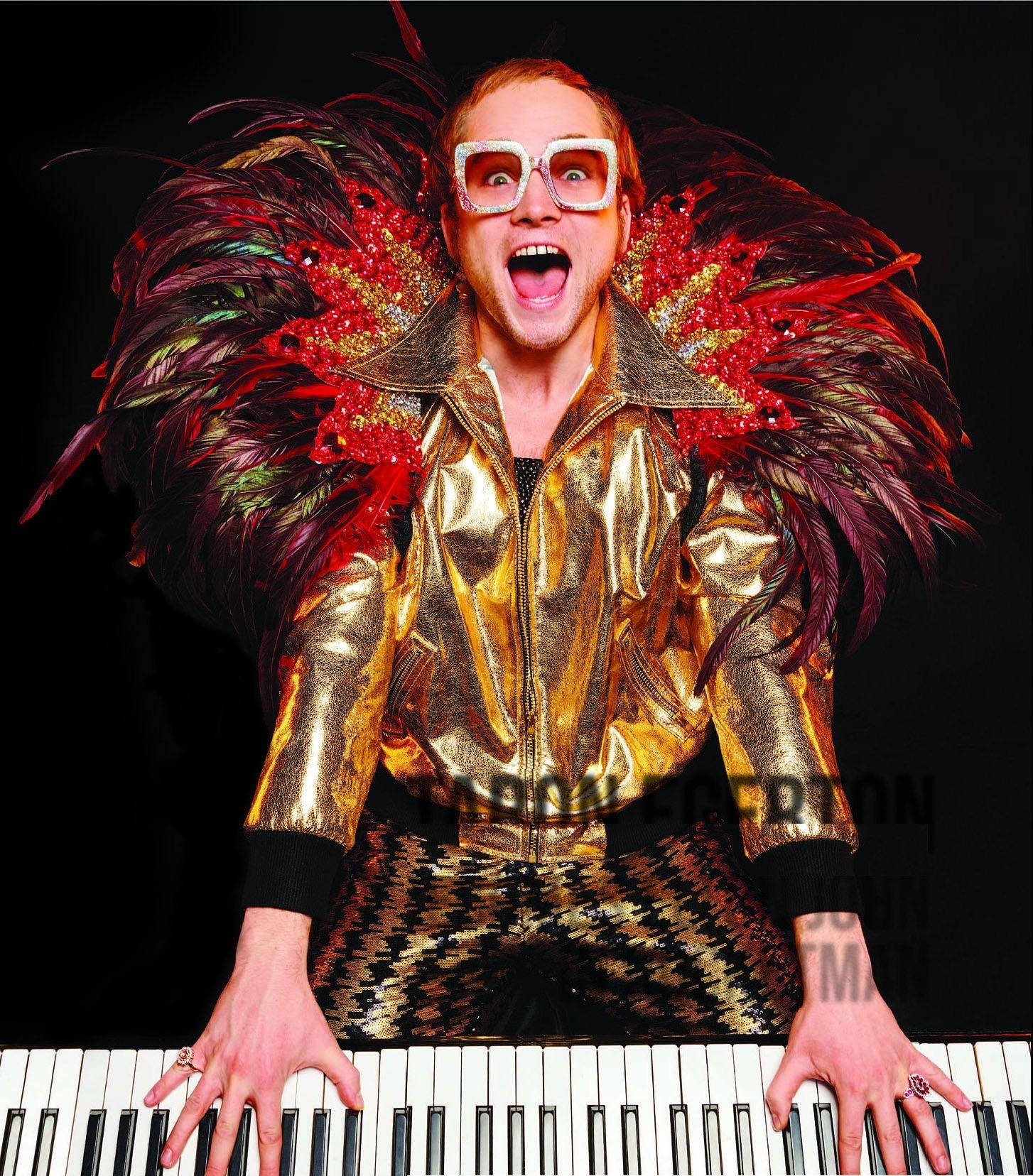In this vibrant and eye-catching portrait-style photograph, Taron Egerton is depicted dressed as Elton John for the biopic "Rocketman." The image captures him from a slightly elevated, frontal perspective as he stands at a piano with both hands placed on the keys, which appear upside down at the bottom of the frame. He sports a striking outfit consisting of a bright, gold reflective jacket adorned with red, burgundy, and green feathers resembling a peacock's plumage, emerging dramatically from his shoulders. The jacket’s collar is embellished with what looks like rhinestones, adding to the flamboyant ensemble. Complementing the jacket, Egerton dons reflective gold and black houndstooth pants, while his bright white, glittery, square-shaped glasses—with a reddish tint—accentuate his look. His hair is neatly cut short, and his mouth is open wide in an expression that conveys both surprise and intense emotion, directed straight at the camera. The background is kept completely black, ensuring that Egerton's dazzling costume and dynamic expression stand out. Rings on each of his hands add a final touch of glitz to this vividly theatrical portrayal.